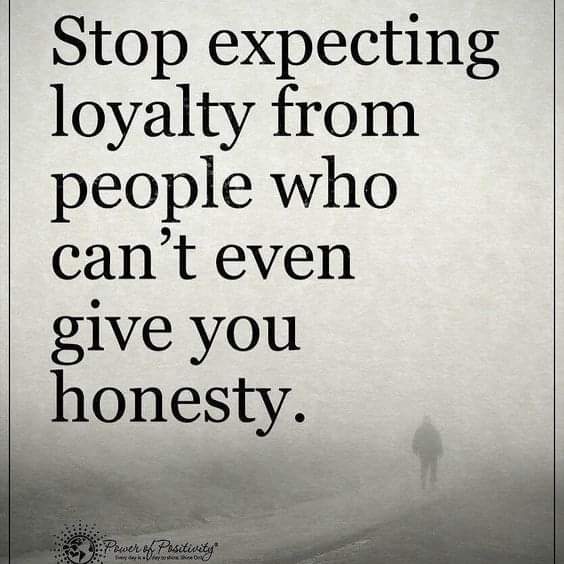The image features a black-and-white, foggy scene with a man walking away on a path in the distance. Bold, capitalized text overlays the center of the image, stating, "STOP EXPECTING LOYALTY FROM PEOPLE WHO CAN'T EVEN GIVE YOU HONESTY." The lettering is arranged in a way that it stands out, with parts of the text trailing vertically down the left side of the poster. Thin gray lines run vertically along both the left and right edges of the image. The lower left corner of the photo includes the phrase "power of positivity" in cursive, accompanied by a logo resembling a black-and-white sun. The scene has a misty atmosphere, enhancing the contemplative mood conveyed by the message.